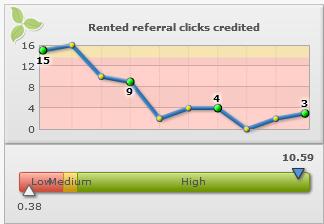The image is a small rectangular snapshot of a computer screen with a gray border and light gray background. Centered at the top, it reads "Rented Referral Clicks Credited" in black text. In the upper left-hand corner, there is a small icon showing three leaves arranged in a circular pattern. Beneath this icon is a line graph with a y-axis labeled in increments of 4, ranging from 0 at the bottom to 16 at the top. The x-axis is unlabeled.

The graph itself shows a downward trend: the blue line starts at 15 on the left, goes down to 9 in the middle, then drops further to 4, and finally reaches 3 at the lower right corner. Green and yellow data points highlight specific values on the line. Below the graph is a horizontal bar divided into three sections: red (labeled "low"), yellow (labeled "medium"), and green (labeled "high"). The green section occupies 80% of the bar, indicating a high status, while the yellow and red sections take up 5% and 15%, respectively. A blue arrow points to "10.59" on the right side of the bar, within the high range, and "0.38" indicated by an arrow on the low end of the bar.